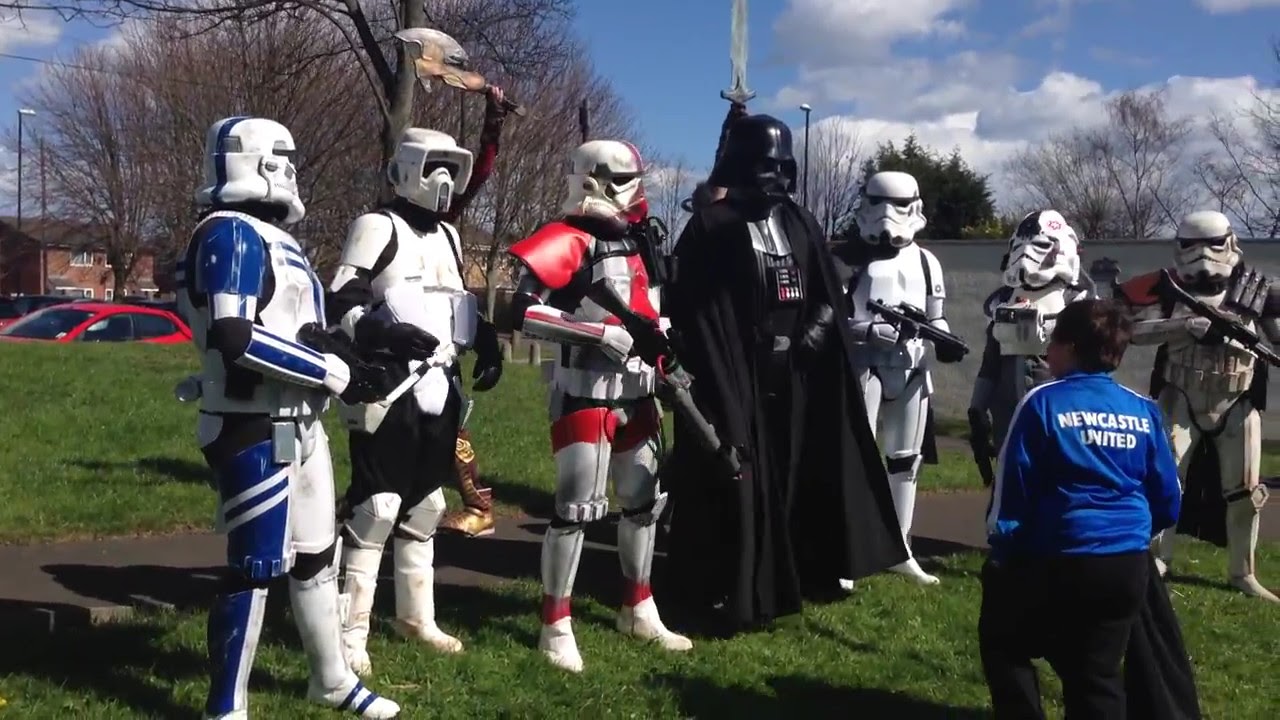In this detailed image, a captivating scene unfolds outdoors on a grassy area. Dominating the middle of the picture stands Darth Vader, intriguingly holding a blaster instead of his trademark lightsaber, surrounded by six individuals dressed up as assorted types of stormtroopers, some adorned with red and blue details on their uniforms. Directly in front of this imposing Star Wars assembly, a person, likely male, is kneeling on the grass with his back to the viewer, donning a distinctive blue Newcastle United jacket. The background presents a suburban setting with sparse trees, bare except for one tree with leaves, flanked by houses and a notable red car partially visible to the left. The clear blue sky dotted with fluffy white clouds adds a serene contrast to the scene brimming with the iconic sci-fi characters. Additionally, a raised sword behind Darth Vader's head further adds to the dramatic ensemble.